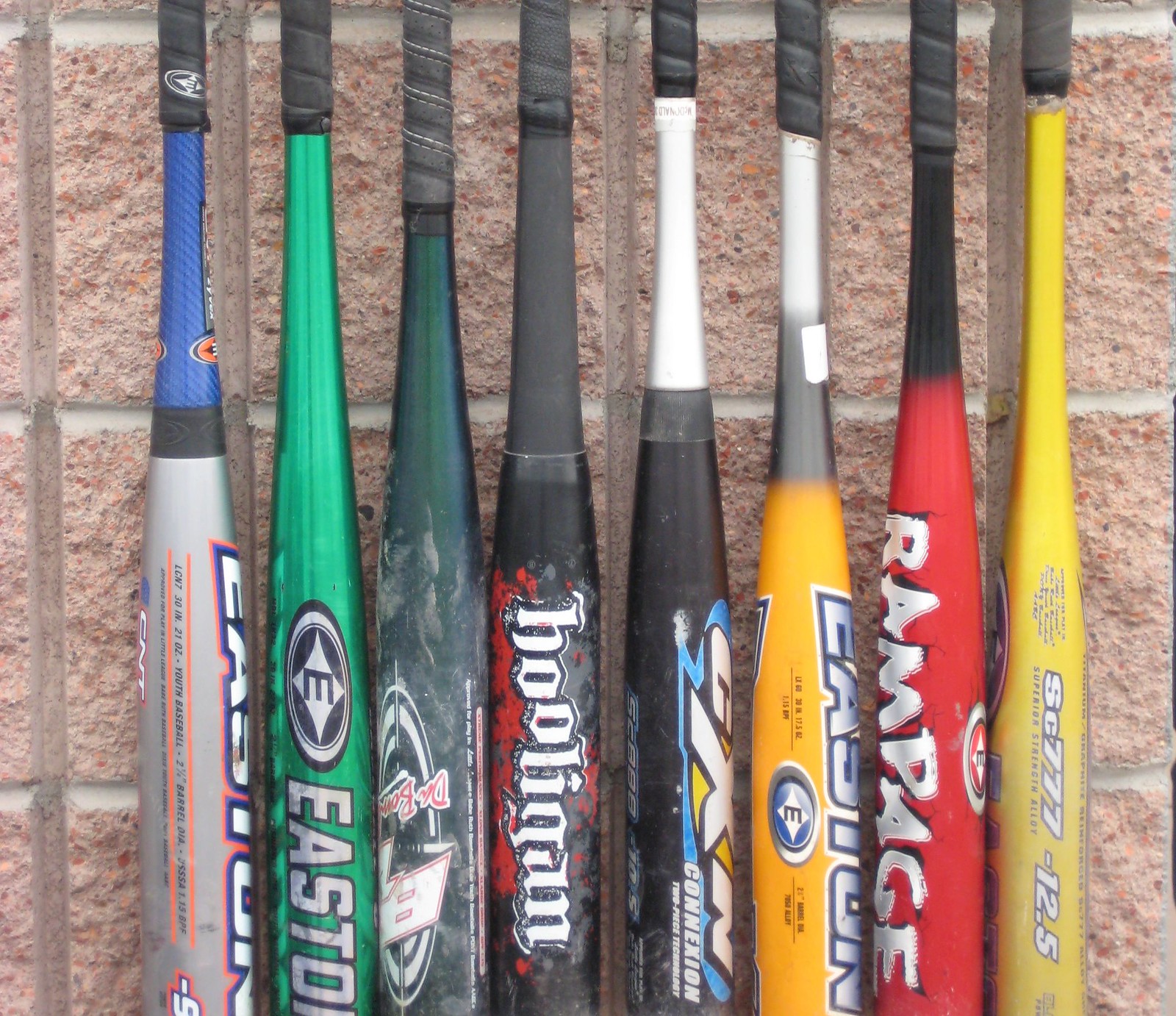This image depicts a lineup of eight baseball bats hanging vertically on a bat rack against a wall that appears to be either stuccoed or tiled to resemble a brick pattern. The wall has a peachy color with speckles of rocks embedded in it. Each bat is positioned with the handle at the top and the barrel at the bottom. 

From left to right, the first bat is a blue and silver Easton. The second bat is metallic green, also an Easton brand. The third bat is a darker green with markings that suggest "Dr." or "Da Bomb." The fourth bat is black with red highlights and says "Hooligan." The fifth bat is black with white, yellow, and blue writing, labeled as "Connection" or possibly "CXN." The sixth bat is yellow with "Easton" written in blue and silver. The seventh bat is red and black with the word "Rampage." The eighth and final bat is yellow and inscribed with "SC777-12.5."

All the bats feature black leather handles where they would be gripped, creating a uniform look despite the variety of colors and brands.